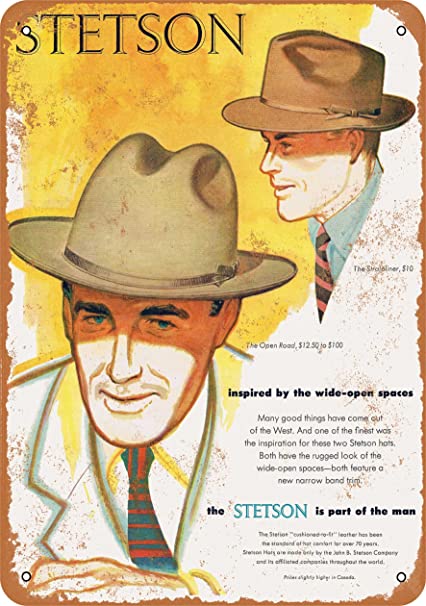The image presents a vintage-style advertisement for Stetson Hats, rendered in portrait orientation with a combination of color illustration, typography, and graphic design. Dominating the ad, "Stetson" is prominently displayed in black outlined font at the top left corner. The background features a splash of yellow, reminiscent of watercolor, framed by a weathered, orange-brown border with rounded edges, enhancing its nostalgic appeal.

At the center left, a dated-looking man gazes upward, dressed in a brown Stetson hat, a suit, and a white shirt. His green and red striped tie adds a touch of color to his attire. Just above him to the right, another man, also adorned in a Stetson hat of a slightly darker hue, looks to the left. He wears a blue (or aqua) shirt and the same green and red striped tie, although a discrepancy in one account mentions a black and orange striped tie. This figure appears from the top of his head to mid-chest, with some parts of his chest and shoulders artistically dropped out.

At the bottom right of the image, black text reads, "Inspired by the wide open spaces, the Stetson is part of the man," emphasizing the intrinsic connection between the Stetson hat and its wearer. The overall composition exudes vintage charm, merging elegant illustration with poignant messaging.